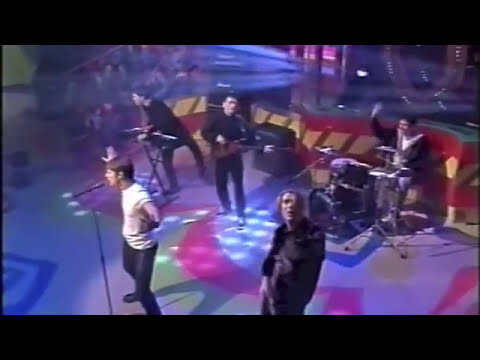The image showcases an old school band in a grainy, low-quality photo, potentially a still from a music video or television show. The stage they're performing on has a vibrant, colorful floor featuring white, red, yellow, and blue shapes and designs. Behind the band is a wall with red and white hues, adorned with several lights. The band consists of five members: the lead singer in a white shirt and jeans, who is singing into a microphone stand; two guitarists, one of whom could be a bass player; a keyboard player positioned to the left; and a drummer in the background. The lead singer is captured with his right hand raised, while the drummer seems to be waving. The scene resembles an old guest show stage, akin to those of David Letterman, Saturday Night Live, or Jay Leno, with an overhead camera angle emphasizing the band's presence slightly to the right on the small, vividly decorated stage.